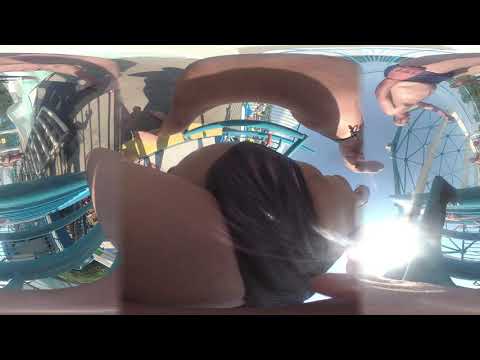The image depicts an outdoor amusement or water park scene captured with a fisheye lens, resulting in a distorted, cluttered view that evokes mixed interpretations. On the upper right corner, a person in a dark suit is sitting with their head between their knees, arms wrapped around their legs, surrounded by green metal bars of an amusement ride, through which a bright white light shines. The central portion features a black piece of cloth with exposed flesh on either side, partially obscured by shadows. The background reveals a mostly blue sky with brown ground below, and a shadowy figure that resembles a person’s face. Additional green bars from the ride and silver metal objects are visible on the far left. The chaotic arrangement of various elements and colors, including blue and brownish-red clutter, along with scattered depictions of water slides, chairs, and other park attractions, contributes to the image’s overwhelming and messy appearance.